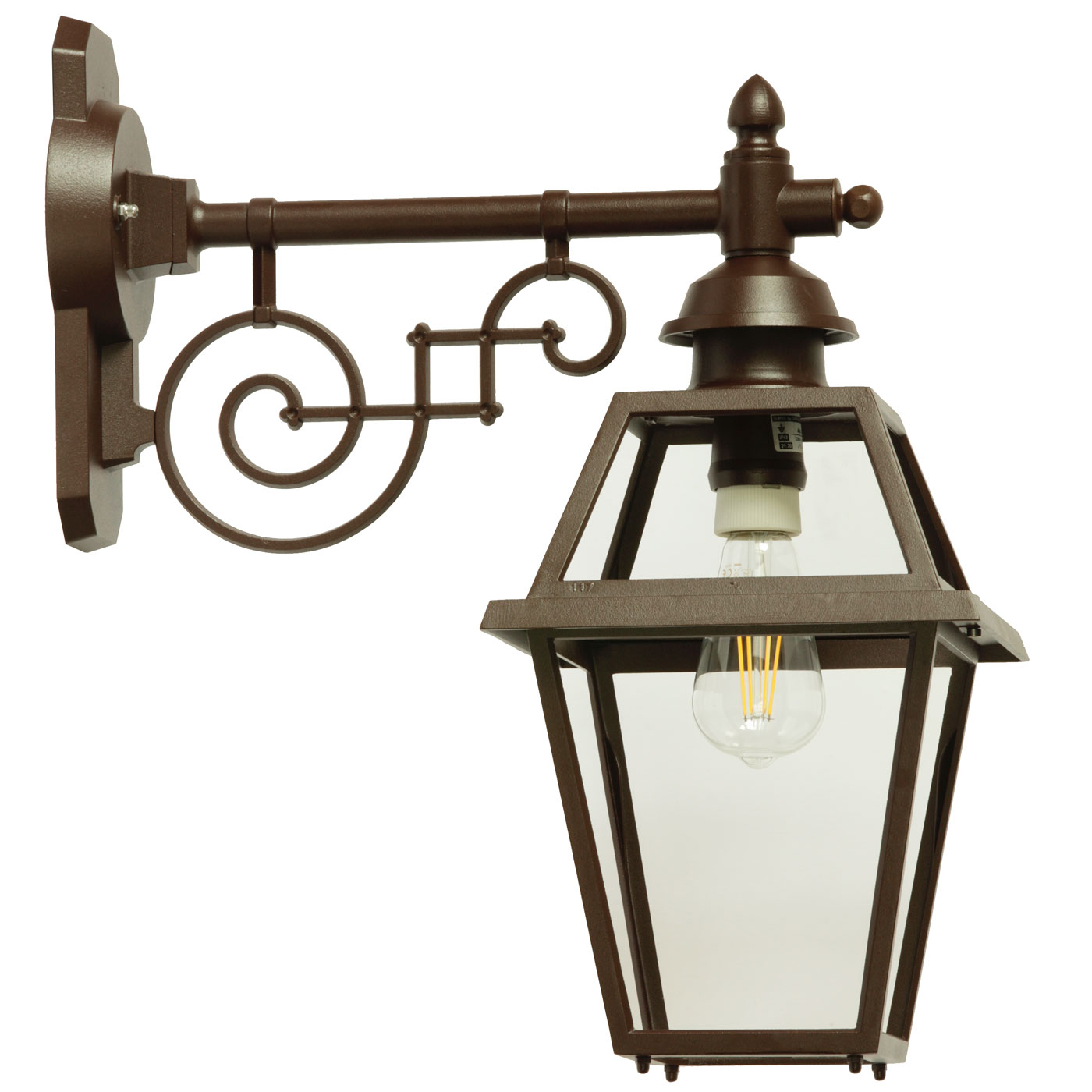The image features an old-fashioned, electric lantern typically found mounted on the side of a house or an outdoor wall. The lantern, designed to evoke a vintage aesthetic, is composed of a brown metal frame with a cage-like structure around the bulb to prevent damage. Its handle boasts intricate, spiral shapes, adding to its charm despite its utilitarian purpose. The bulb inside appears to be a classic filament style or designed to mimic an old-timey appearance, emitting a warm yellow glow. The overall setting and presentation suggest the image could be part of an advertisement or product catalog, with the lantern depicted in isolation against a plain background, devoid of any mounting pole or wall. The photo is primarily monochromatic, featuring shades of black, white, and the yellow illumination from the bulb.